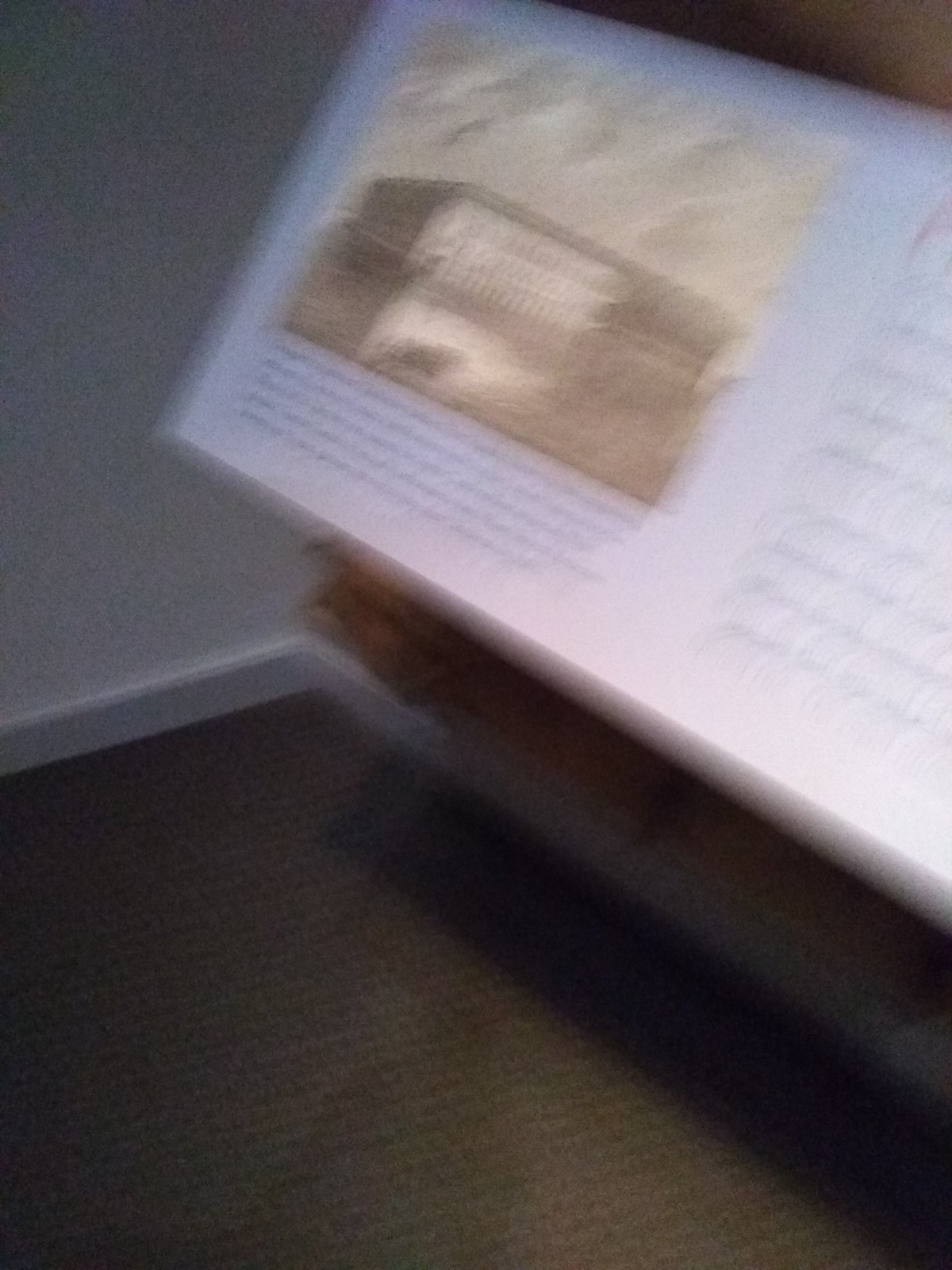The image captures a highly blurry scene, likely taken in a moment of motion, featuring what appears to be an informational display typically found in museums or art galleries. The display is angled, suggesting it serves to describe a diorama or exhibit within the space. However, the setting is perplexing: the room's corner is visible, showing a carpeted floor and a gray wall with baseboards, elements more characteristic of residential interiors than public exhibition spaces. Despite the poor focus and movement blur, the upper portion of the image maintains the appearance of a professional museum or gallery description panel, while the lower part hints at a public display setup. The incongruity between the residential-like flooring and baseboards with the museum-style angled display adds a layer of uncertainty to the scene's true nature.